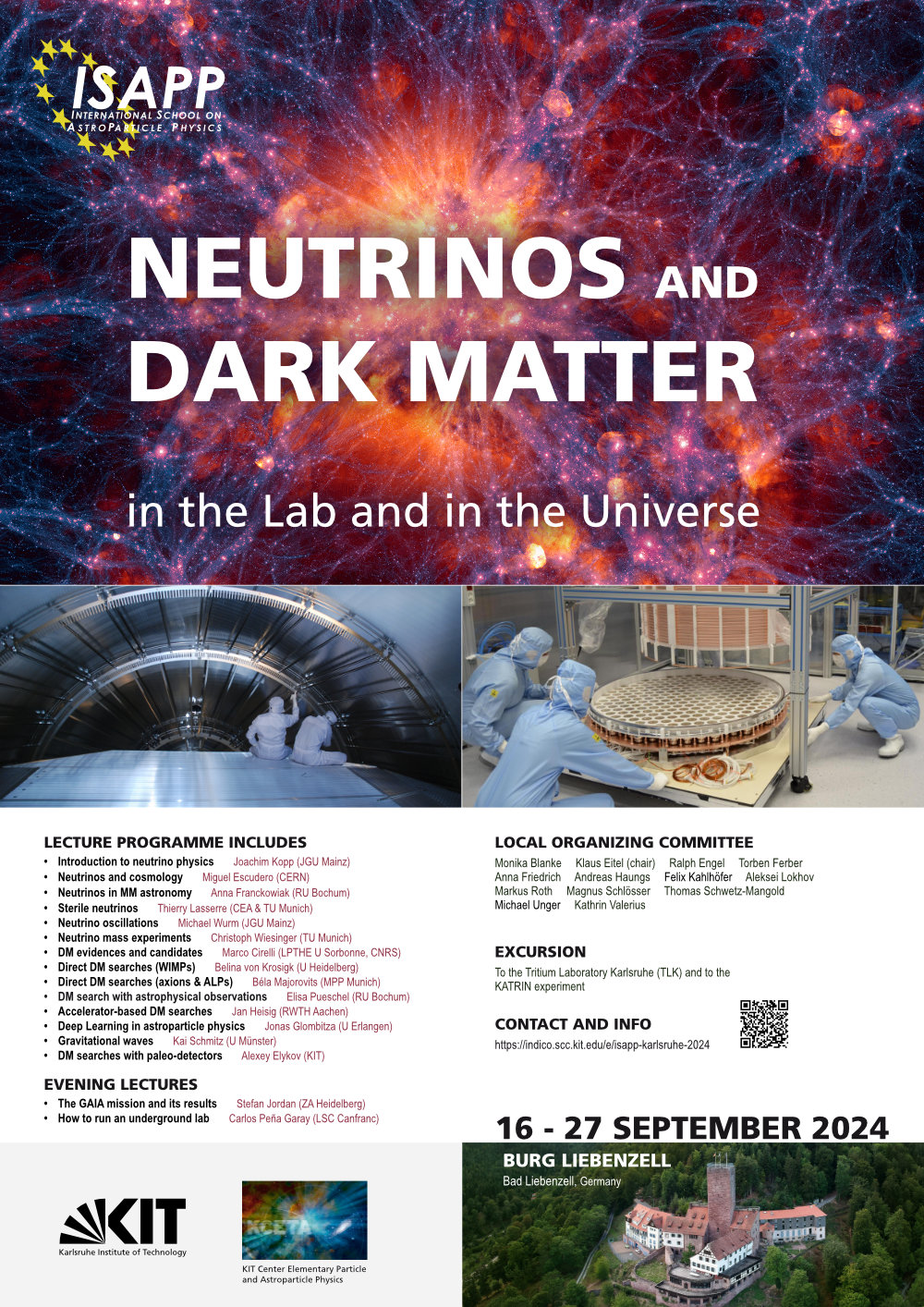The flyer for the "International School on Astrophysical Physics (ISAPP)" advertises a lecture series titled "Neutrinos and Dark Matter in the Lab and the Universe," scheduled to take place from September 16th to 27th, 2024, in Berg Liebenzell, Germany. The top of the flyer features a vivid image of a colored supernova, creating a striking backdrop. Dominating the center in large, bold white text from POSON, the theme of the lecture is clearly presented. Beneath this header, there are two photographs depicting laboratory settings. In one image, scientists are seated in a dome-like structure, which could be part of a particle accelerator. In the other, several researchers are gathered around a circular device, possibly a photon collector or scientific sensor. The lower section of the flyer outlines the lecture program, detailing various topics and speakers, along with additional information about the local organizing committee, excursions, and contact details. A small QR code is also provided for further information or registration.